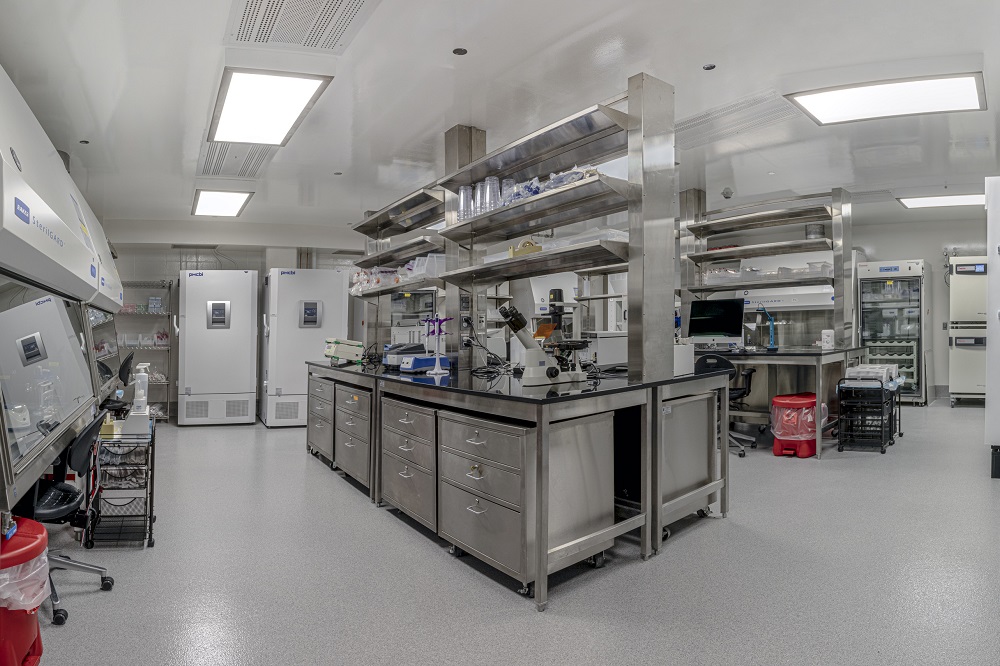The photograph depicts the interior of a sterile scientific or medical laboratory situated in what appears to be a basement due to the absence of windows and the presence of fluorescent lighting. Central to the image is a large stainless steel work table with several shelves extending from the floor to the ceiling, stacked with various laboratory equipment, glassware, and other scientific instruments. Prominently on the main workspace sits a microscope and additional machinery, indicative of activities such as DNA analysis. Beneath this workspace are multiple stainless steel filing cabinets for storage. To the right is another work area featuring a computer chair and a large monitor, flanked by industrial computer equipment. Both sides of the room have red biohazard bins, emphasizing the laboratory's meticulous attention to safety and cleanliness. The overall environment is marked by shiny white floors and ceilings, reinforcing the sterile, high-tech atmosphere necessary for precise scientific work.